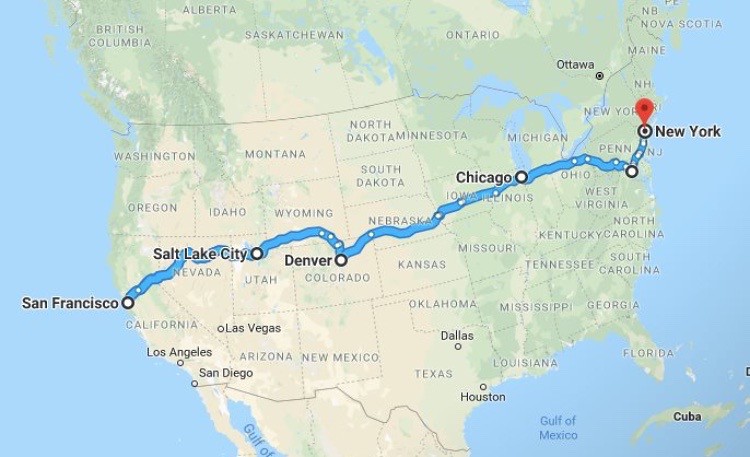This is a screenshot of an older version of Google Maps displaying the continental United States. The map prominently features a thick blue line indicating a route that starts in San Francisco, marked with a bold label. The route proceeds eastward, highlighting several major cities along the way: Salt Lake City, Denver, and Chicago. The blue line continues until it reaches New York, where it terminates with a red, bulbous drop pin. This pin signifies the endpoint of the route, confirming that the journey begins in San Francisco and concludes in New York. The map effectively illustrates a cross-country route from the west coast to the east coast of the United States.